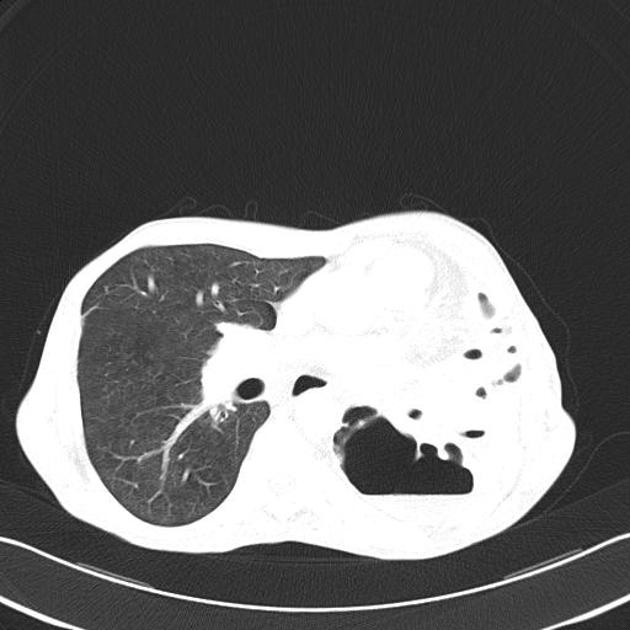This image is a black-and-white MRI scan showcasing a potential cross-section of a brain or kidney. The square picture features a predominantly black background, especially towards the upper part. The central area of the image is mostly white with various shades of gray, highlighting internal structures that may indicate different tissue densities. On the left side, there's a distinct white mass with a dark gray, kidney-shaped area inside it, which could indicate a notable feature or abnormality. The bottom right of the image contains a blank, jet-black area, enhancing the contrast. Additionally, there are two curved lines, one thicker and black, and the other thinner and white, that move from left to right and could represent anatomical separations or boundaries. The image lacks any timestamps or labels, making specific identification challenging for non-experts.